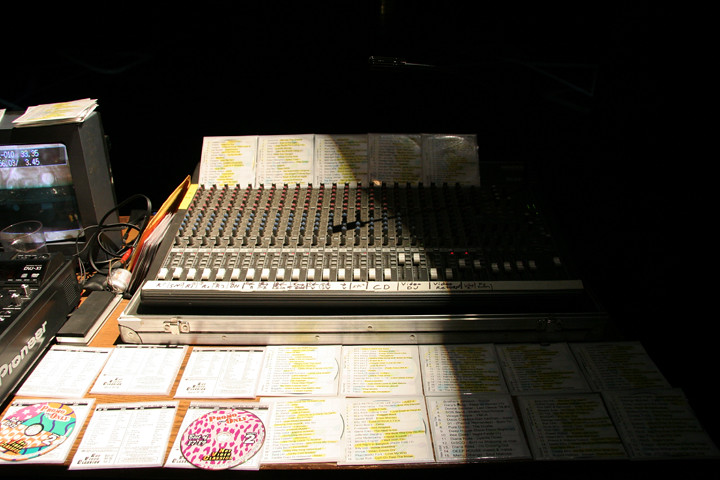This image depicts the inside of a vintage radio station or DJ's workspace, likely dating back to the 1970s. Dominating the scene is a brown wooden table cluttered with several CDs and handwritten track listings, many of which are highlighted in yellow. Central to the image is a soundboard, featuring a myriad of buttons and controls essential for audio mixing. On the left side, a black piece of equipment with the brand name 'Pioneer' prominently displayed in white, suggests the presence of a video or recording device. The background of the image fades into black, offering no visible details beyond the immediate setup. This carefully curated, old-fashioned space with its characteristic handwritten notes and highlighted tracks starkly contrasts with the modern, computer-driven studios of today.